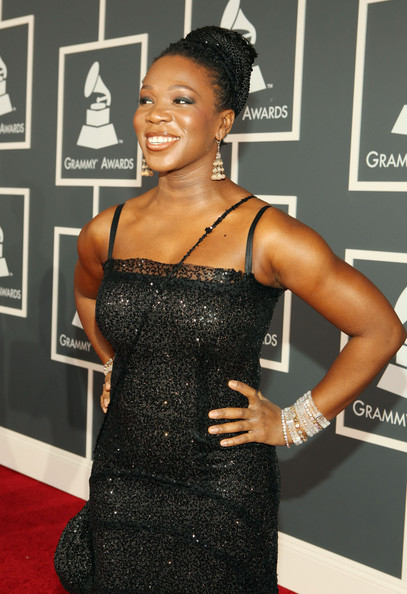At the Grammy Awards, an elegant African American woman stands radiant on the red carpet, framed by a backdrop adorned with the Grammy Awards logo. The logo, featuring rectangular boxes with phonographs and the words "Grammy Awards," is scattered in two rows across the grayish background. With her hair styled in an updo, she exudes confidence as she looks slightly to her right, her bright smile capturing the moment. She wears a stunning black sequined dress with narrow shoulder straps and delicate lace detailing at the chest. Complementing her look, she accessorizes with a series of sparkling bracelets on both wrists, long dangly earrings, and a matching black purse. Her fit, muscly arms and the glitzy details of her attire make her the focal point of this glamorous scene.